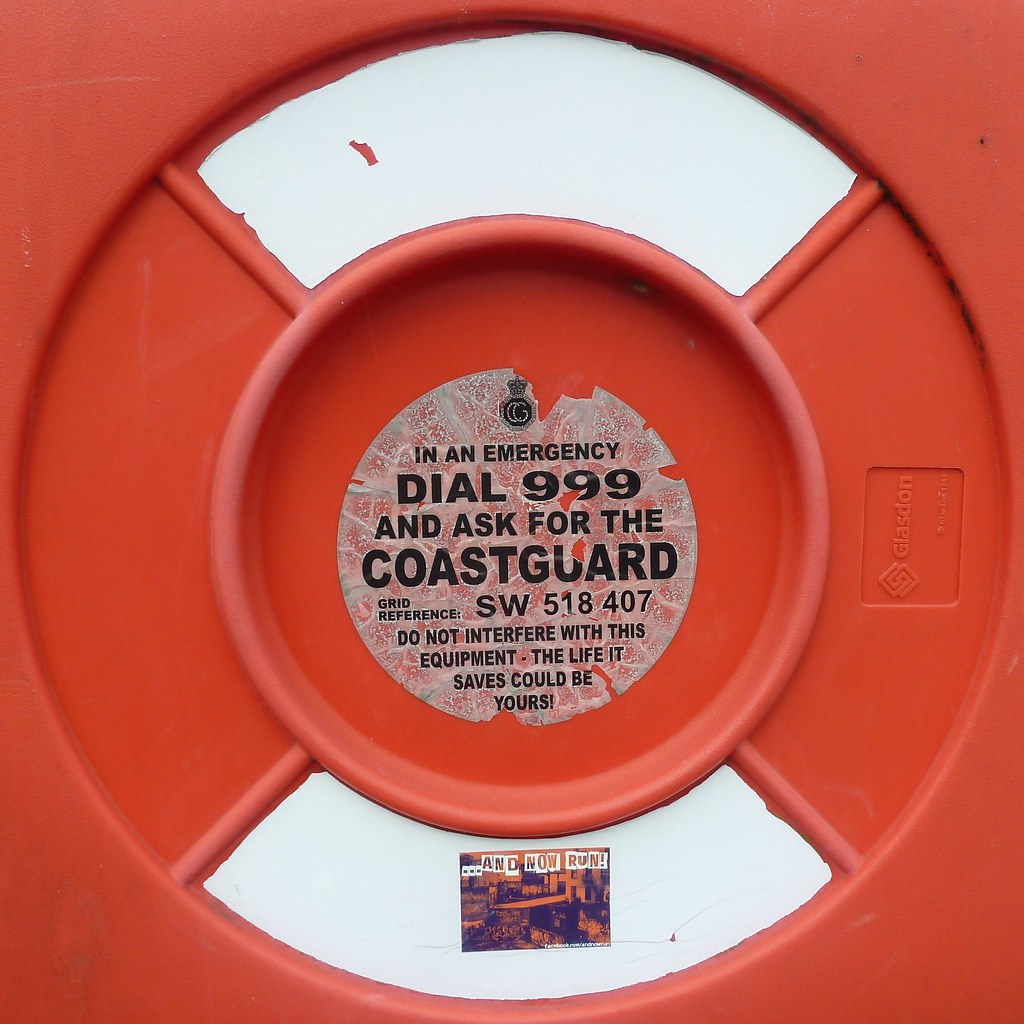The image depicts a bright orange plastic sign with a prominent circular design in the center, divided into four sections. The top and bottom sections of the circle are white, while the left and right sections are orange. Inside the circle, a detailed decal is present, slightly peeling, which reads: "In an emergency dial 999 and ask for the Coast Guard. Grid reference SW518407. Do not interfere with this equipment. The life it saves could be yours," all in black text. At the very top of this decal is a small crown emblem, hinting at a British or European origin. Below this central message, in the bottom white section, there's a sticker that reads "and now run," adorned with orange and black graphics. To the right section of the circle, there's a logo that says "Glaston." The entire design, with its vibrant colors and critical emergency instructions, closely resembles a life preserver, emphasizing its function and importance in maritime safety.